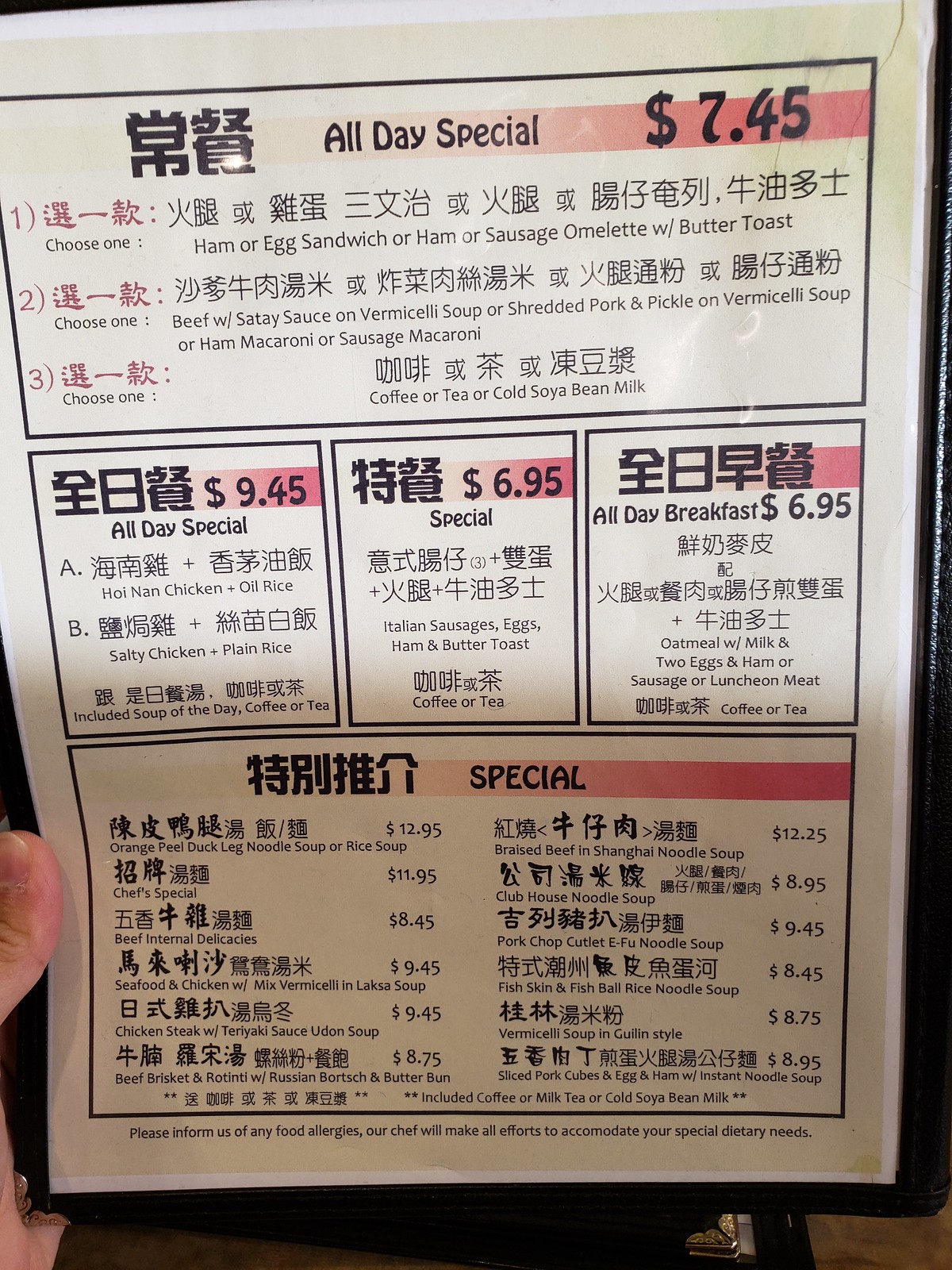The photograph captures a white menu held by a light-skinned person, with the menu encased in a plastic sleeve and framed by what appears to be a black leather or faux leather border. The menu takes up nearly the entire vertical rectangular frame, with the person’s thumb and part of their palm visible in the lower left corner, grasping the item. The menu itself features predominantly Chinese characters with occasional English text, sectioned into five distinct areas each bordered in black. The top horizontal section is labeled "All Day Special $7.45," while the bottom horizontal section is labeled "Special." The central strip consists of three square boxes: the leftmost labeled "All Day Special $9.45," the center "Special $6.95," and the right "All Day Breakfast $6.95." The text throughout is in black, with thin red banners behind some of the prices and labels, extending from the upper right corners of their respective sections.